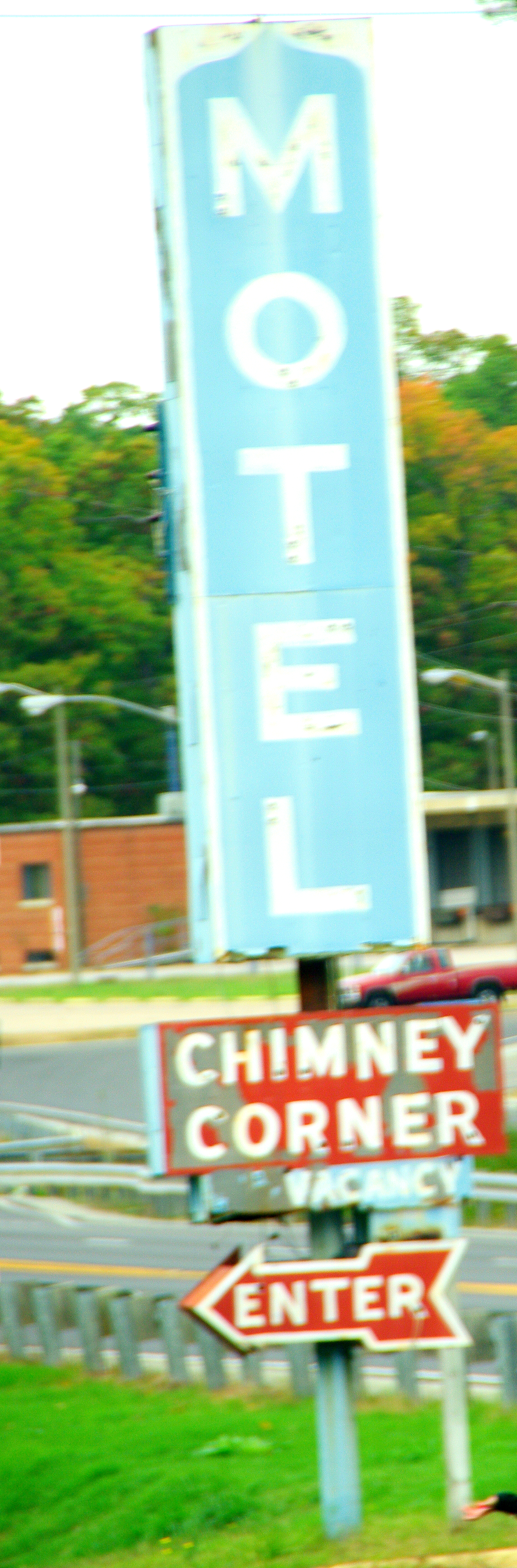A vertical, weathered sign stands prominently in the image, its once vivid colors now faded by time. The top portion of the sign features a blue background with white letters spelling out "MOTEL." Below it hangs a rectangular, horizontal sign with remnants of red paint, bearing the name "CHIMNEY CORNER" in white lettering. Just beneath this, a red arrow bordered in white points to the left, accompanied by the word "ENTER" in white letters, suggesting it may have been a neon sign at some point. The photograph is taken during the day, making it difficult to ascertain if the sign lights up at night.

In the background, a highway can be seen, cutting across the frame and adding to the atmosphere of a roadside stop. Under the sign, lush green grass hints at the rural or suburban setting. Further in the distance, an orange, two-story brick building adds a touch of architectural interest, standing quietly behind the sign and contrasting against the sky. The overall scene depicts a nostalgic slice of Americana, capturing the essence of a bygone era.